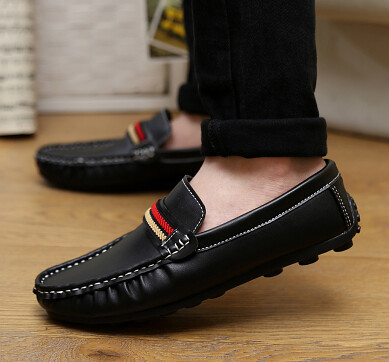This photograph captures a detailed close-up of a pair of black slippers or moccasins, resembling penny loafers. The slippers are adorned with white stitching along the edges and feature a band across the top embellished with curly fabric in red, yellow, and black stripes. The heels of the moccasins have flat, nylon-like spikes. The image showcases the wearer, possibly a man or a boy, who is dressed in black pants rolled up slightly at the bottom and is standing barefoot on a light-colored wooden floor with visible wood grain. The left foot is prominently displayed while the right foot appears slightly out of focus in the background. A white wall can be seen in the image's backdrop.